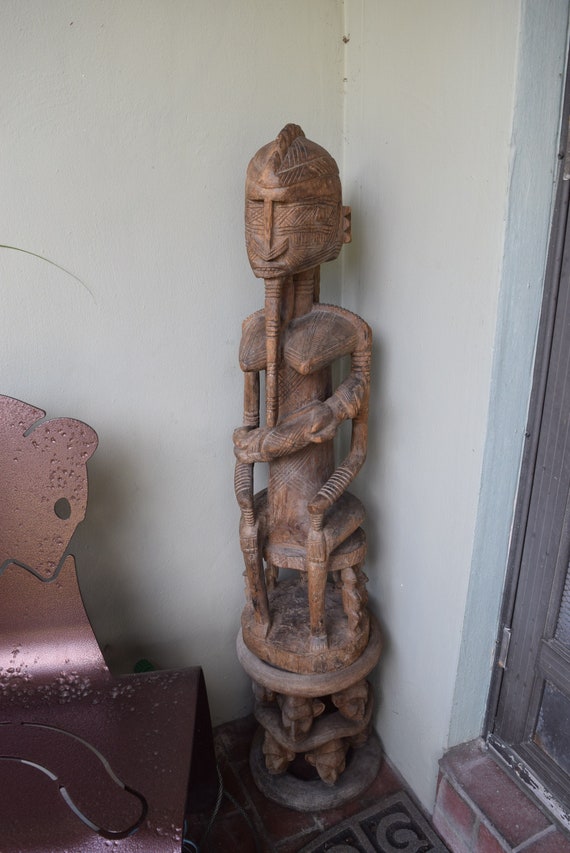The photograph captures an ancient African wooden sculpture of a seated female figure placed in the corner of a room with white walls and a shut door visible to the right side of the image. The sculpture, detailed with chiseled features and a long nose, sits on a chair with a circular base. The figure exudes an intense expression and appears to have elongated, slender arms, which are adorned with bracelet-like cuts around the wrists. Adjacent to the sculpture, on the left side of the image, is a thinly pounded piece of copper metal and a single blade of grass peeping out. The setting distinctly blends elements of ancient African art in a modern indoor environment with notable contrasts such as a dark scratch on the wall and light filtering in from outside, creating an intriguing juxtaposition.